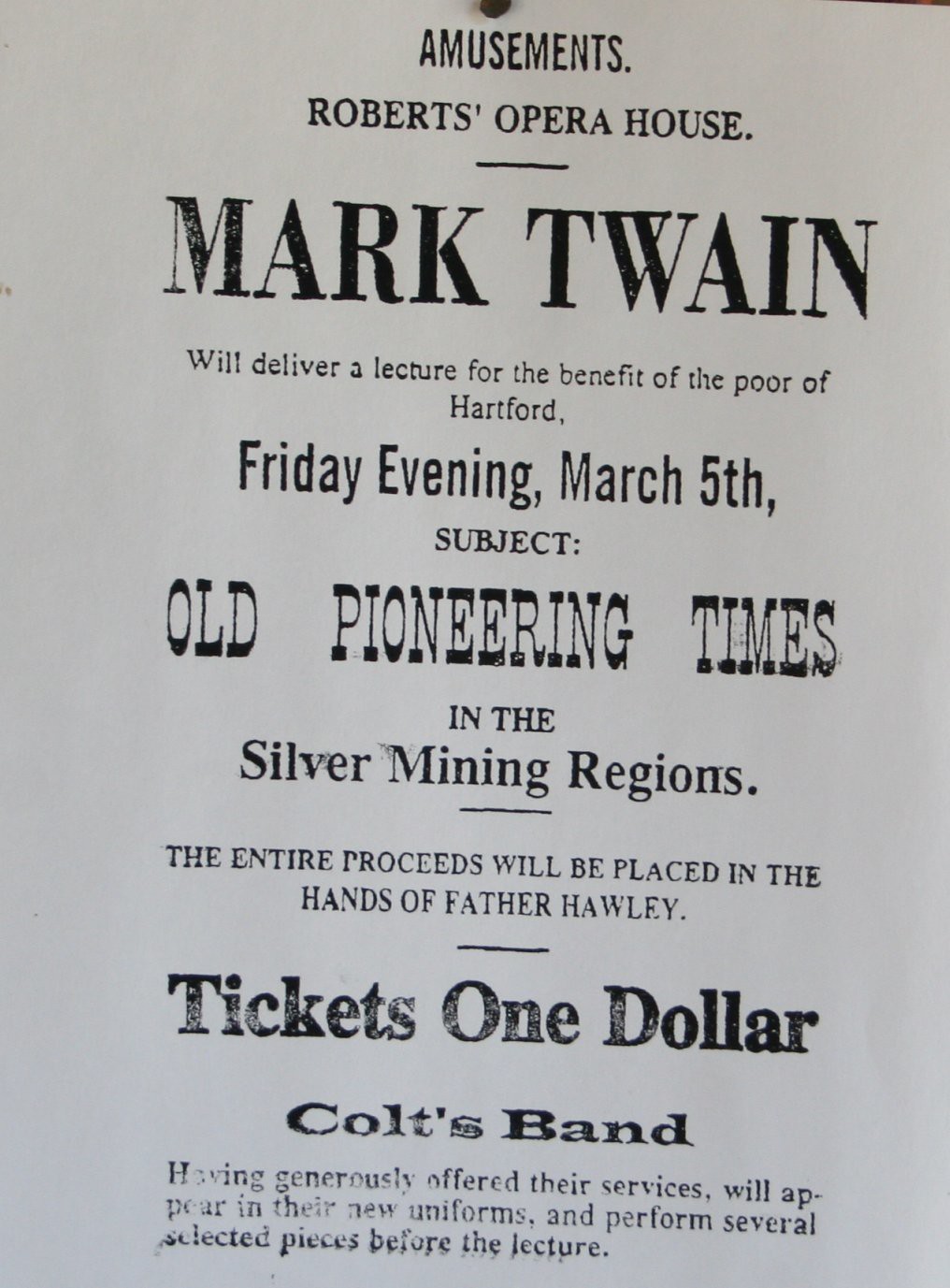The photograph showcases an old black-and-white announcement, likely a flyer or sign, from Roberts Opera House. At the top, it prominently features the heading "Amusements" followed by "Roberts Opera House." Beneath these titles appears the name "Mark Twain" in large, bold text, indicating his participation in the event. The flyer details that Mark Twain will deliver a lecture on Friday evening, March 5th, with the subject being "Old Pioneering Times in the Silver Mining Regions." The lecture is held for the benefit of the poor of Hartford, with all proceeds administered by Father Hawley. Additional information indicates that tickets are priced at one dollar. Notably, the Colts Band, having generously offered their services, will don new uniforms and perform several selected pieces before the lecture. The entire flyer is in simple black ink on a white background, with a mix of large and small fonts lending it an authentic, old-timey feel.